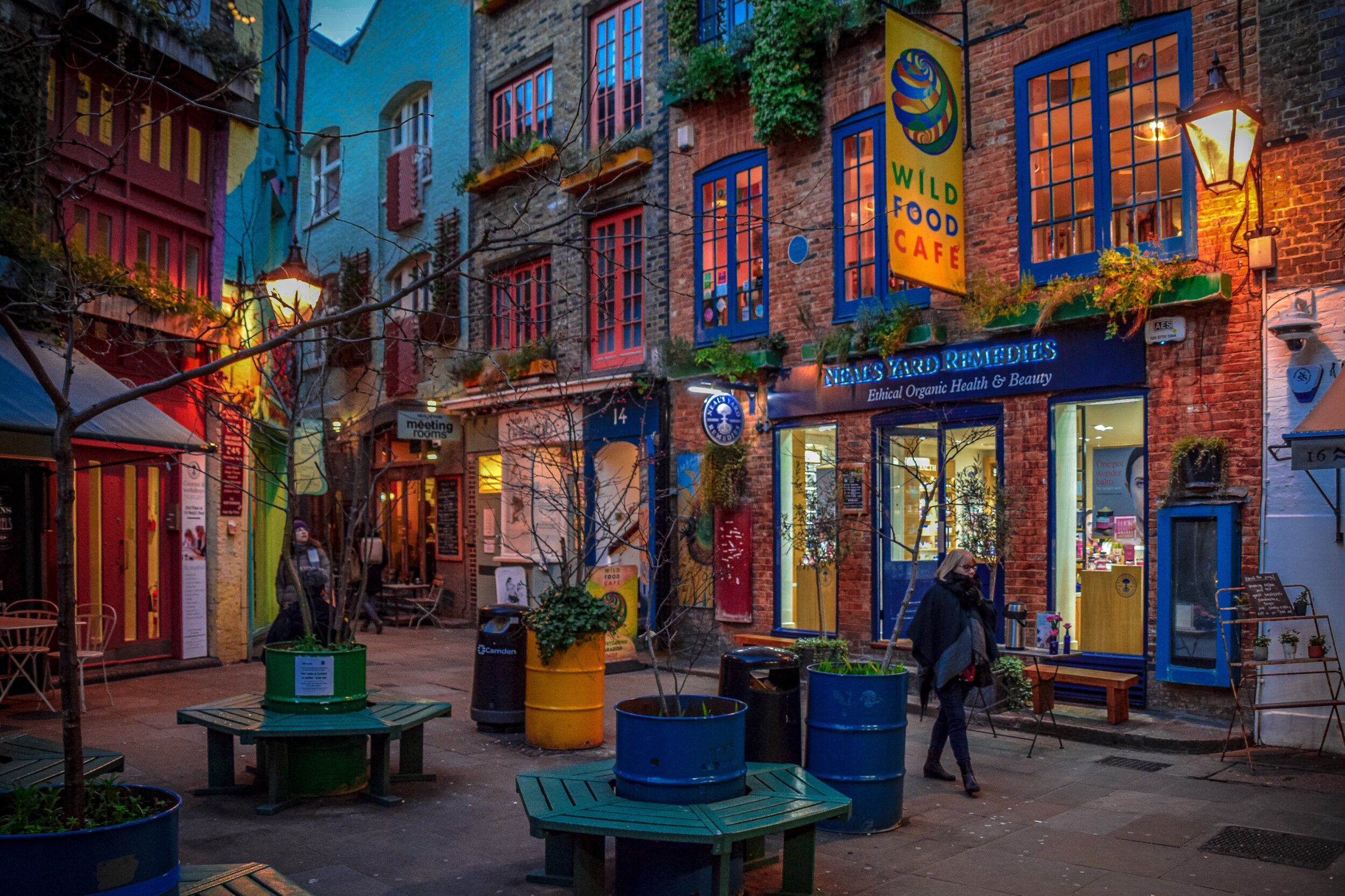In this highly realistic painting, which almost resembles a photograph, we see an evening scene of a vibrant small-town area. Dominating the foreground are three-story brick buildings, their facades illuminated by glowing storefront lights. The building closest to us displays a sign for "Wild Food Cafe," while another shop features blue text indicating "Neal's Yard Remedies." Windows on the second level of the buildings emit a warm reddish-yellow light, adding to the cozy evening atmosphere. 

A blonde woman in a black coat with a scarf walks along the sidewalk, passing by storefronts with lined tables showcasing beauty products or perfumes. In the middle of the scene, where two rows of buildings meet, hexagonal benches surround a central circular spot filled with plants. Additional splashes of color are provided by four barrels—one blue, one yellow, and two dark-colored—now serving as planters along with a nearly-bare tree to the left. 

The streetlights are lit, casting a serene glow over the area, while a mix of red, blue, and yellow doors add an extra layer of vibrancy to this lively scene. Despite the realistic details, the painting captures an almost magical quality of this bustling small town in the evening.